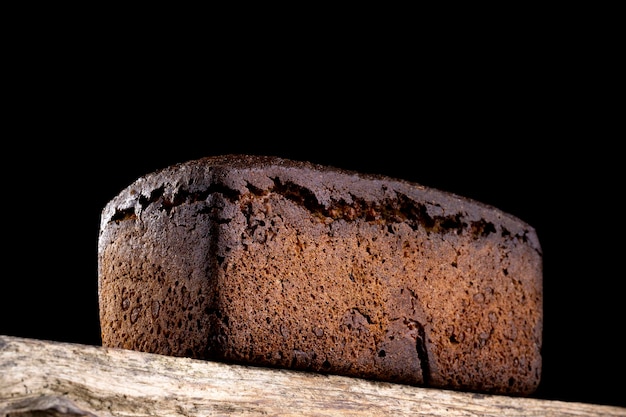The image is a color photograph of a single, uncut loaf of bread resting on a rough, worn wooden surface. The background is pitch black, providing a stark contrast to the loaf and the table. The bread, rectangular in shape, appears slightly burnt with a very dark, almost black crust on the top. The sides are a lighter, rusty brown color, with several darker patches contributing to its rugged appearance. The top of the loaf is notably crackly, hinting at its overcooked nature, with cracks running around the perimeter. The bread sits on a piece of unpainted, unsanded, and possibly warped wood that serves as a makeshift table or countertop, accentuating the rustic and unrefined look of the overall setting.